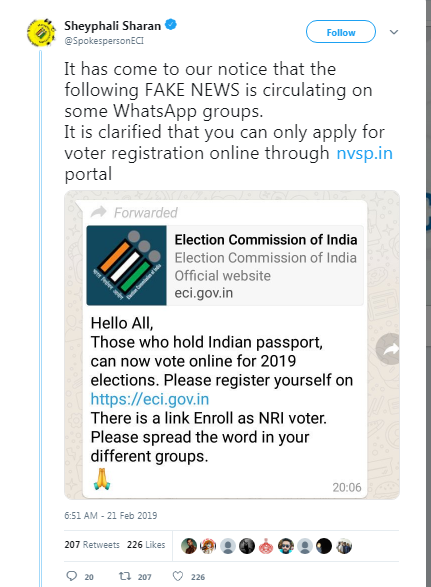Screenshot of a social media post purportedly from Sheyphali Sharan, the Spokesperson for the Election Commission of India (ECI) (not confirmed if Facebook). The header includes a white "Follow" button with a blue outline and font, alongside a downward-facing menu.

The post alerts users to the circulation of fake news on WhatsApp groups, clarifying that voter registration for Indian elections can only be done online through the official portal NVSP.in, which is provided as a clickable blue link.

The message states:
"It has come to our notice that the following fake news is circulating on some WhatsApp groups. It is to clarify that you can only apply for voter registration online through NVSP.in."

The official notice from the Election Commission of India further reads:
"Hello all, those who hold an Indian passport can now vote online for the 2019 elections. Please register yourself at ECI.gov.in."

The links provided are highlighted in blue, indicating their clickable nature. The note ends with a call to action, urging users to share this information with their contacts.